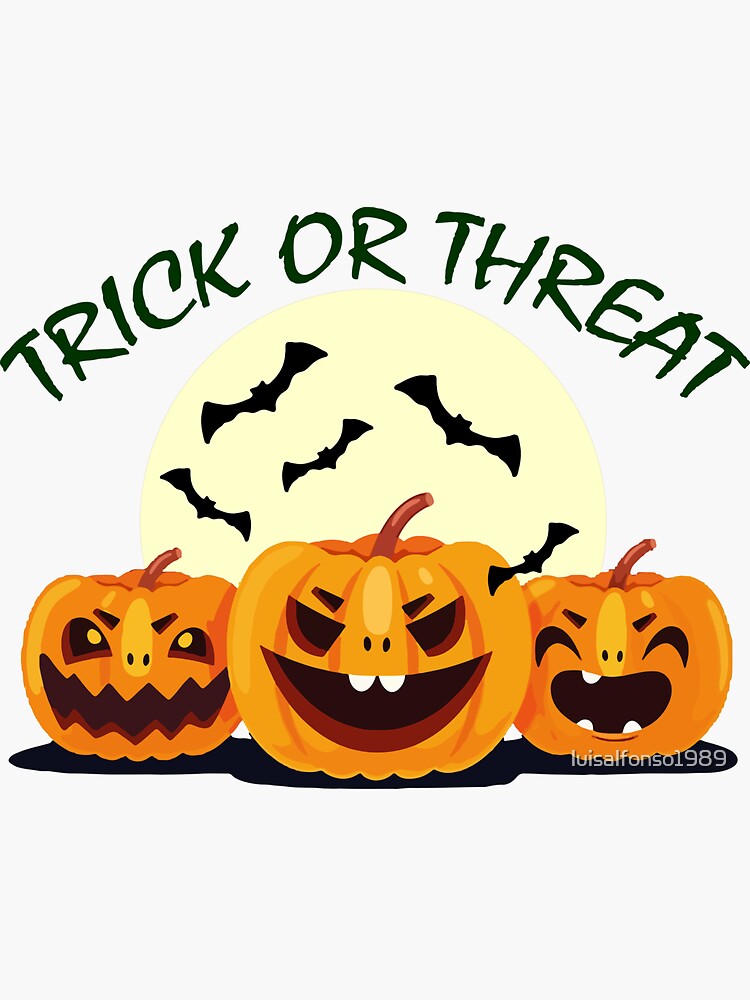The rectangular artwork, with its dimensions being twice as long on the sides as the top and bottom, features a set of three smiling, cartoonish orange pumpkins, each exhibiting a different expression. The pumpkin on the left has semi-circle eyes and a mouth with sharp fangs, topped with a brown stem. The middle pumpkin is adorned with two white buck teeth and also has a brown stem. The third pumpkin displays three teeth, two on the bottom and one on top.

Centered in the composition is a yellow circle encircled by black outlines of bats, and above the circle is the black text "Trick or Treat." The background is a light gray, which enhances the elements of the artwork. Notably, on the lower right side of the image, there is additional text that reads "Louisol Fonsole 1989." This digital artwork blends playful Halloween imagery with a subtle, eerie feel, through the pumpkins’ mischievous expressions and the surrounding bats.